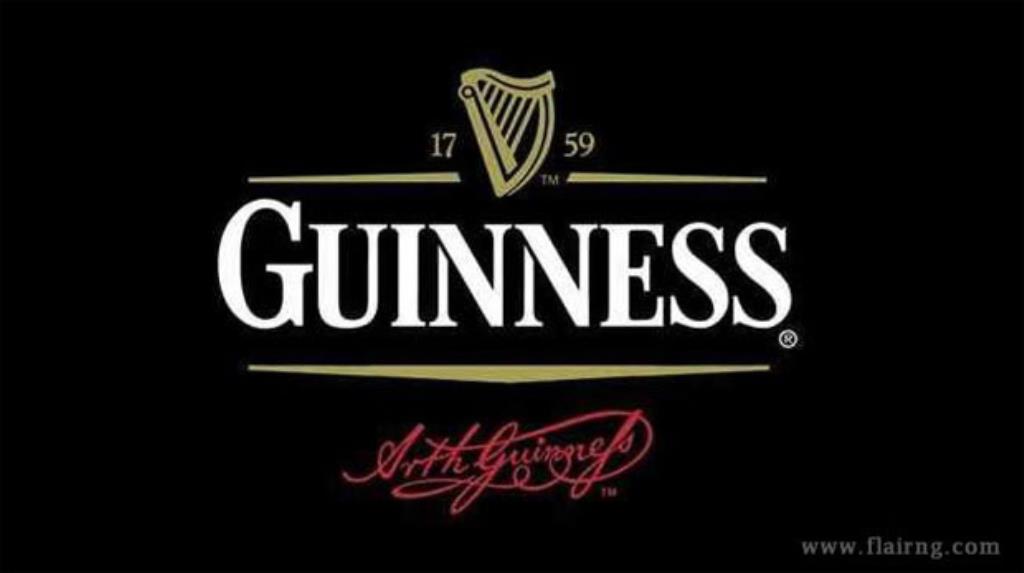This is an advertisement featuring the Guinness Beer Company logo. The prominent elements are centrally aligned against a black background. At the top, there is a golden harp with the numbers "17" and "59" on either side, symbolizing the year 1759. Below the harp, a gold trademark symbol can be seen. The main section displays the word "Guinness" in large, white, Times New Roman-style font, with a particularly oversized "G." Flanking the central text are two horizontal gold bars, the top of which is broken at the center to accommodate the harp. Underneath the "Guinness" text sits a reserved symbol. Toward the bottom of the advertisement, the signature "Arth Guinness" is written in red cursive script, surrounded by decorative red squiggly lines. Finally, in the bottom right-hand corner, the URL "www.flareng.com" appears in small, light gray letters.